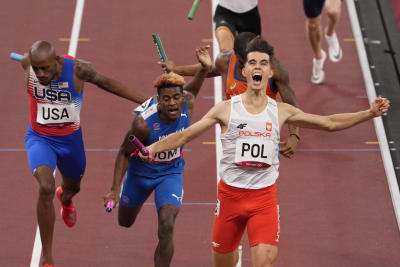In the photo taken near the finish line of a relay race, a jubilant Polish runner with brown hair is seen celebrating his victory. He is wearing a white tank top with the letters "P.O.L." on it and red shorts, and he is holding a pink baton. He is facing the camera with his arms outstretched in celebration. Closely behind him are two other runners. To his left is a black athlete from the USA, identifiable by his blue, white, and red uniform emblazoned with "USA" and holding a blue baton. One of his competitors, dressed in a blue uniform, is slightly obscured but visible next to him. In the background, two more runners are partially visible; one is wearing a white shirt and black pants, and the other has black pants and white shoes. The scene captures the thrilling and competitive spirit as the runners approach the finish line on a track and field course.